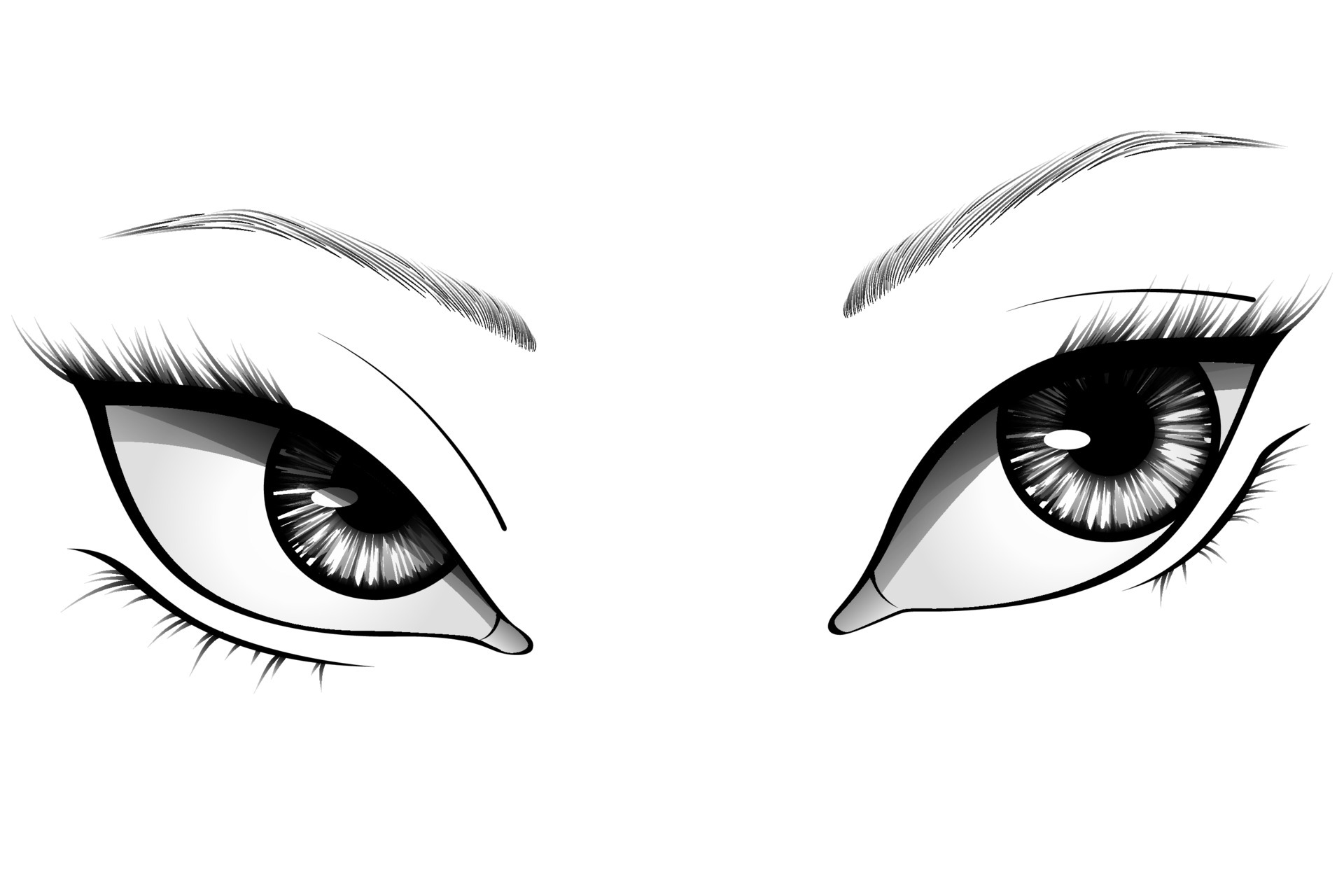This illustration is a meticulously detailed black and white depiction of a pair of eyes, likely those of a woman, with slanted, almond shapes. Each eye features well-defined tear ducts in the bottom corners, adding to their expressive quality. The irises are a sparkly grey, with specks of white radiating around the black pupils, creating an illusion of depth and light reflection. The whites of the eyes are immaculate, enhancing the vivid appearance of the gaze directed towards the viewer.

The eye's outlines are adorned with prominent, lengthy upper lashes and shorter, spaced lower lashes, giving a feathery, delicate touch. The upper lashes show some light wisps, adding to the intricacy of the artwork. Two fine lines, representing the natural creases of the eyelids, provide further realism and shadowing to the scene. Above these eyes, the arched and very thin eyebrows are crafted with fine black strokes, contributing to the overall refined and elegant composition of the piece.